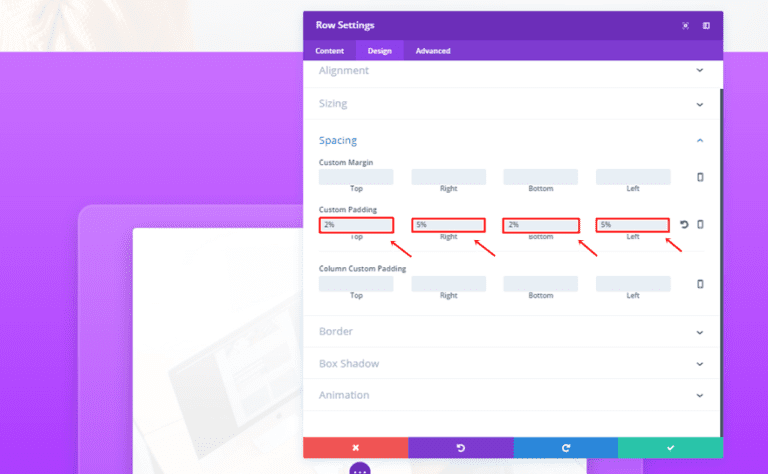A screenshot featuring a user interface with a predominantly purple background. At the top of the interface is the header "Role Settings." Below this, there are tabs labeled "Content," "Design," and "Advanced," with "Design" highlighted against a light purple rectangle. Within the "Design" section, there are various customization options for "Alignment," "Sizing," and "Spacing." The "Spacing" category is selected, indicated by a blue highlight.

Within the "Spacing" section, there are options for adjusting "Custom Margin" and "Custom Padding," with input areas for adjusting margins at the "Top," "Right," "Bottom," and "Left." Specific values are set as follows: Top: 2% (enclosed in a rectangle), Right: 5% (in a rectangle), Bottom: 2% (in a rectangle), and Left: 5% (in a rectangle). Each input area also has a red arrow pointing to it for emphasis.

Further down, there are additional options for adjusting "Column Custom Padding" with the same top, right, bottom, and left settings available. Below these, there are additional customization options for "Border," "Box Shadow," and "Animation." The image likely originates from a photo editing application.